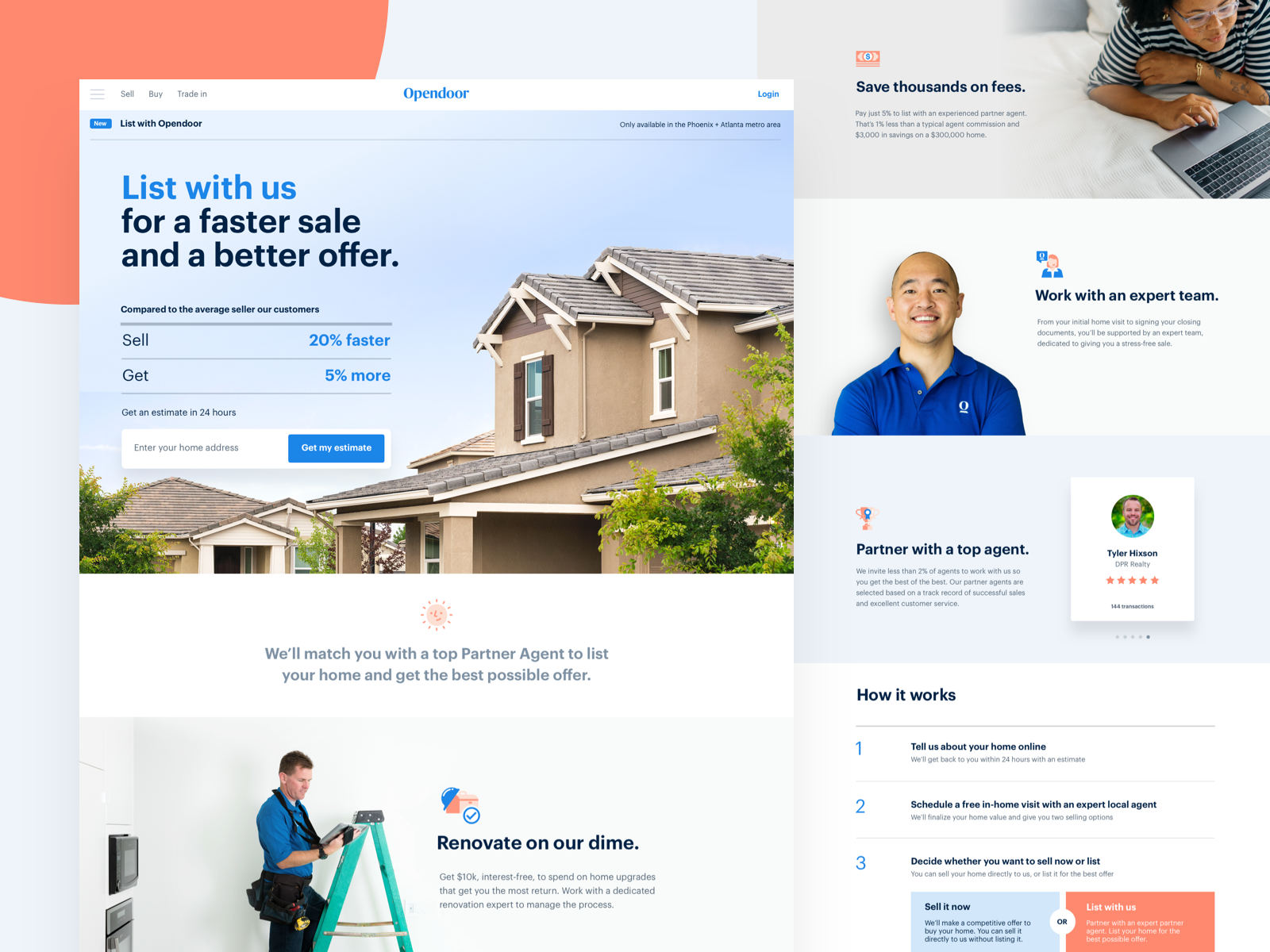**Detailed Caption:**

The website showcases a comprehensive real estate or home listing service. The primary background features the main homepage, filled with various informational blurbs detailing the service offerings. Dominating the visual is a prominent pop-up window that draws immediate attention. The pop-up displays an inviting image of a house under a clear blue sky, with the focus on the top section of the house's front porch awning and second-story windows, accompanied by ample space filled with fluffy clouds to the left.

The foreground text on the pop-up stands out, highlighting promotional messages such as "List with us for a faster sale and a better offer," promising a 20% faster sale and 5% higher offers. The message encourages users to sign up, likely by entering their email, to access this streamlined service.

Surrounding the main ad, the website outlines detailed information about its functionality. It emphasizes that users will be paired with a top partner agent to secure the best possible offer for their home, and assistance with renovations will be provided. The information is visually supported by a collage of various images that represent different aspects of the service, contributing to a holistic presentation of what the platform offers.